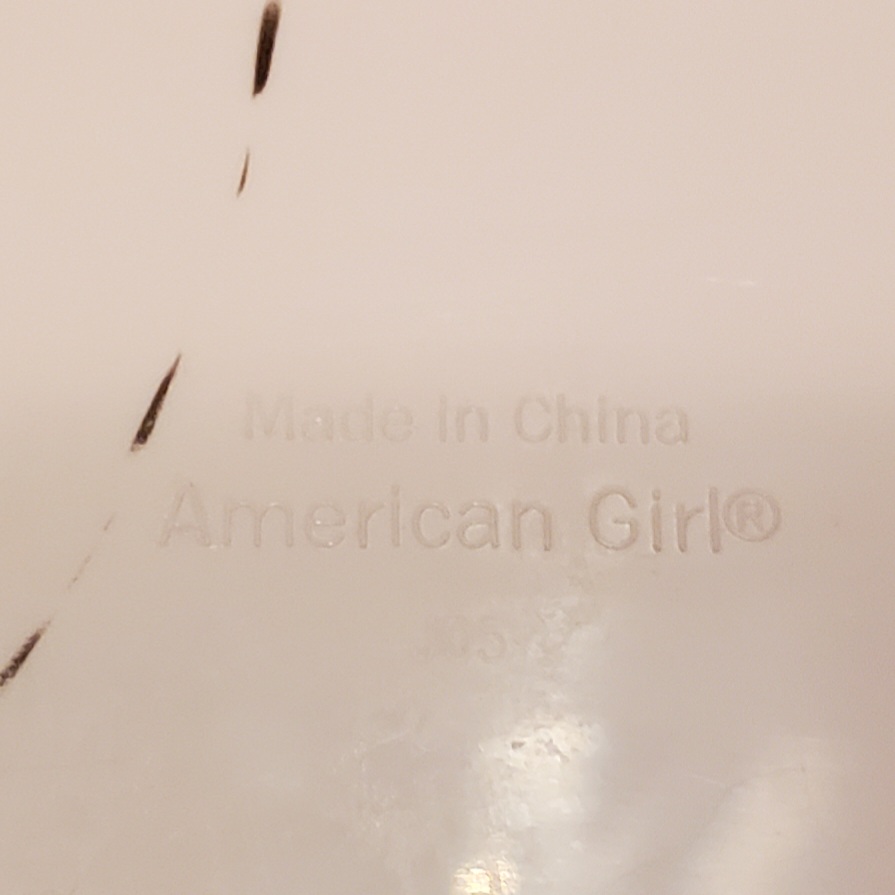This image showcases a porcelain or ceramic item, predominantly cream in color. Notably, about a third of the way from the top, a distinct brown dotted line is featured. The dots are spaced significantly apart and curve downwards, approaching the bottom left-hand side. The item is engraved with the phrase "Made in China," indicating its origin. Additionally, the brand "American Girl" is stamped on it, along with a small registered trademark symbol (®). Light reflects subtly off the bottom surface, adding a soft gleam to the photograph. At the center of the piece, there is a series of numbers, although they appear quite faded; the last digit is clearly a five, while the preceding digit seems to be a zero.